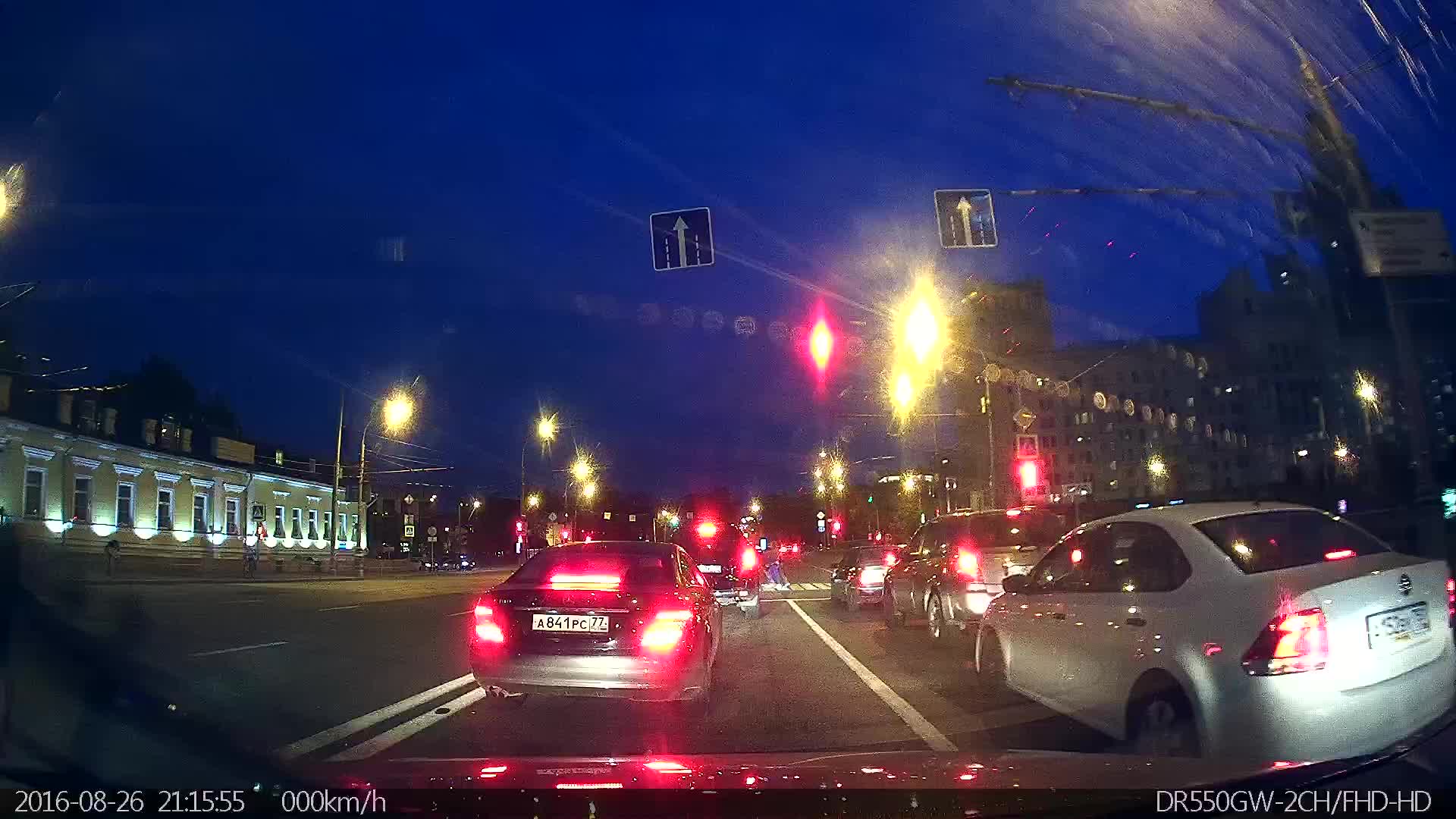A nighttime image capturing a modern European dashboard-mounted camera on a highway. The scene is set in the late evening, with the sky transitioning to night. The license plates, distinguishable as non-U.S., suggest the location is in Europe. Multiple vehicles are visible, including at least one clearly identifiable SUV and possibly another, with three cars' brake lights illuminated. Directional arrows are marked on the road, which features both stationary and seemingly free-floating signs. On the left, there are buildings and a section of highway devoid of traffic, adding depth to the picture.